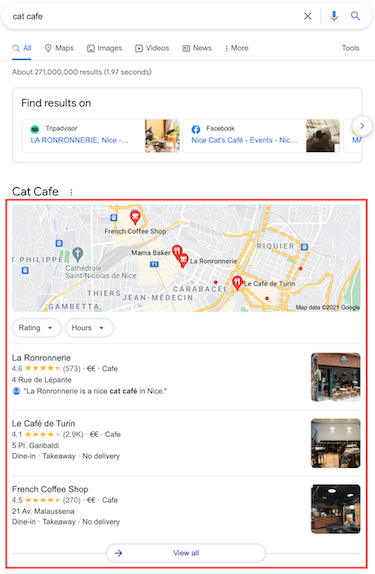The screenshot displays the results of a Google Maps search for "Cat Cafe," prominently showing the search query at the top. The map interface reveals several highlighted locations marked with red icons. Directly beneath the map, users can sort results by ratings and hours. The search yields approximately 271 million results, with detailed information on three specific cat cafes in France.

1. **Le Grand Reinnere** - Located in Nice, this café boasts a rating of 4.6 stars and is described as a lovely cat café. Three accompanying images show a charming, cozy interior likely to appeal to cat enthusiasts.

2. **Le Café de Turand** - This café has a 4.1-star rating and offers dine-in and takeaway services, but no delivery. The images suggest a welcoming atmosphere.

3. **French Coffee Shop** - With a 4.5-star rating, this café also offers dine-in and takeaway services, excluding delivery. Its ambiance appears similar and equally inviting.

This map section is distinctly outlined in red, directing focus to these prominent options while above it, alternative platforms like TripAdvisor and Facebook offer additional related searches.